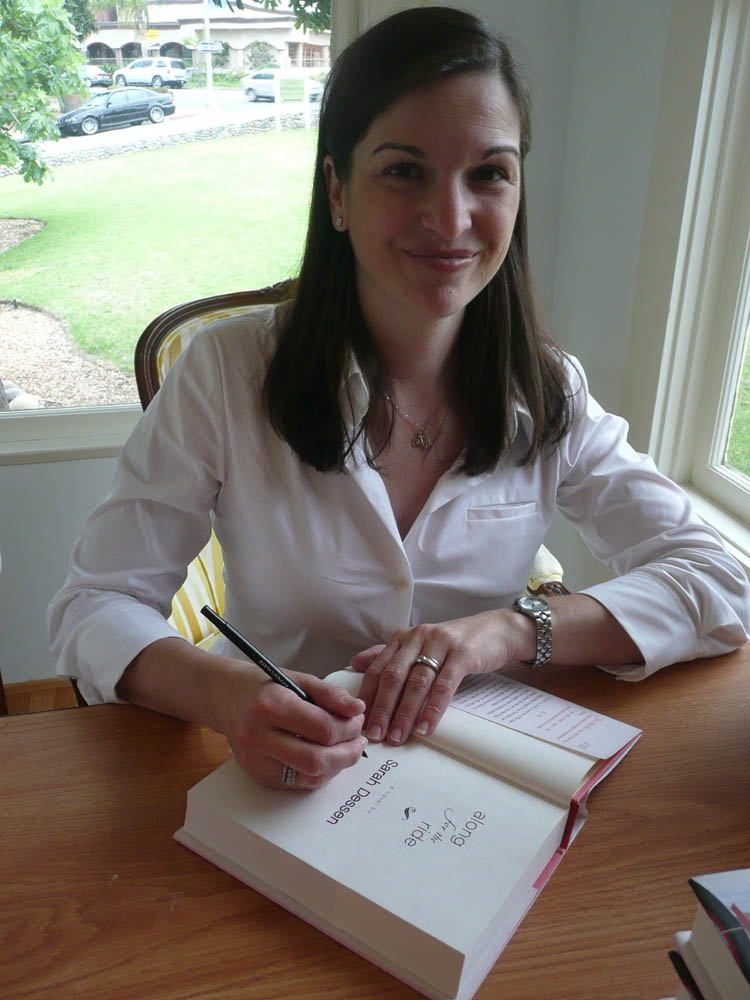In the image, a woman, likely in her mid to late 30s with straight brown hair that cascades just past her shoulders, is seated at a brown-topped desk, signing a book titled "Along for the Ride" by Sarah Dessen. Clad in a white blouse buttoned just below the neck and adorned with a necklace, she has a slight smile on her face as she engages in the book signing. The woman is accessorized with diamond earrings, a gold watch on her left wrist, and rings on both hands, including her left ring finger. Holding a Bic black pen in her right hand, she appears poised to autograph either the cover or the inside of the book. Over her right shoulder, a window reveals a backdrop featuring trees, cars, and a hint of houses, indicating it is daytime. This setting suggests a book signing event, with the woman—presumably Sarah Dessen herself—connecting with her readers.